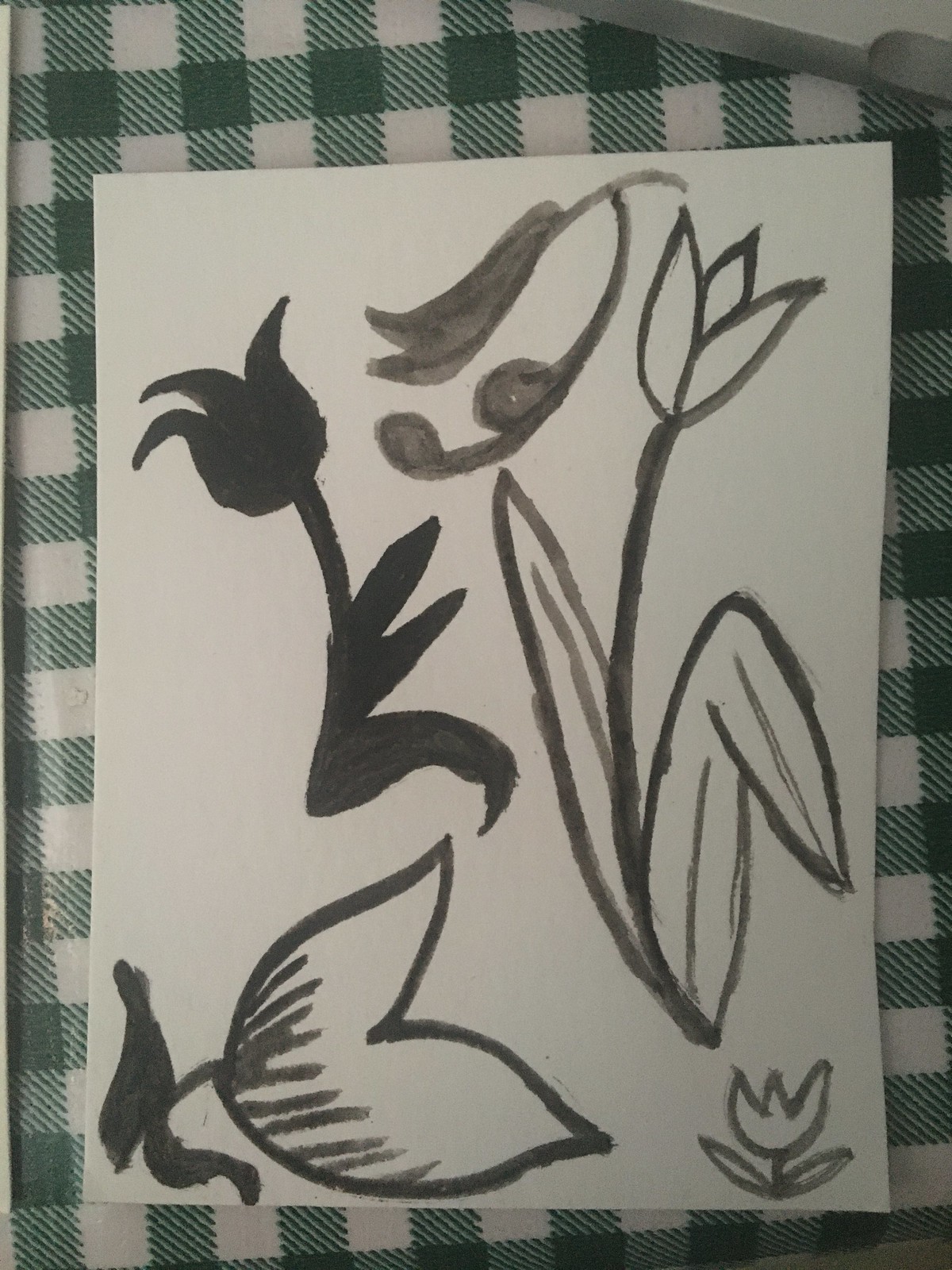This is a photograph of a monochromatic drawing or painting, likely done by a child, on white paper. The artwork features four separate tulip-like flowers done in various shades of black and gray, each with distinct characteristics and dimensions. One flower is entirely filled in black, while the others are rendered in lighter grays and black outlines. The flowers are distributed across the paper: a large tulip bending to the right with wide leaves, a smaller tulip in the lower right corner with oblong leaves forming a V-shape, another bold-stroked tulip with stripes in the lower left corner, and a centrally placed tulip with a segmented head and curved leaves. The white paper nearly fills the frame of the photograph, which includes a background of a hunter green checked tablecloth or kitchen towel. The artwork is unsigned and there are no textual markings indicating the time or date it was created.